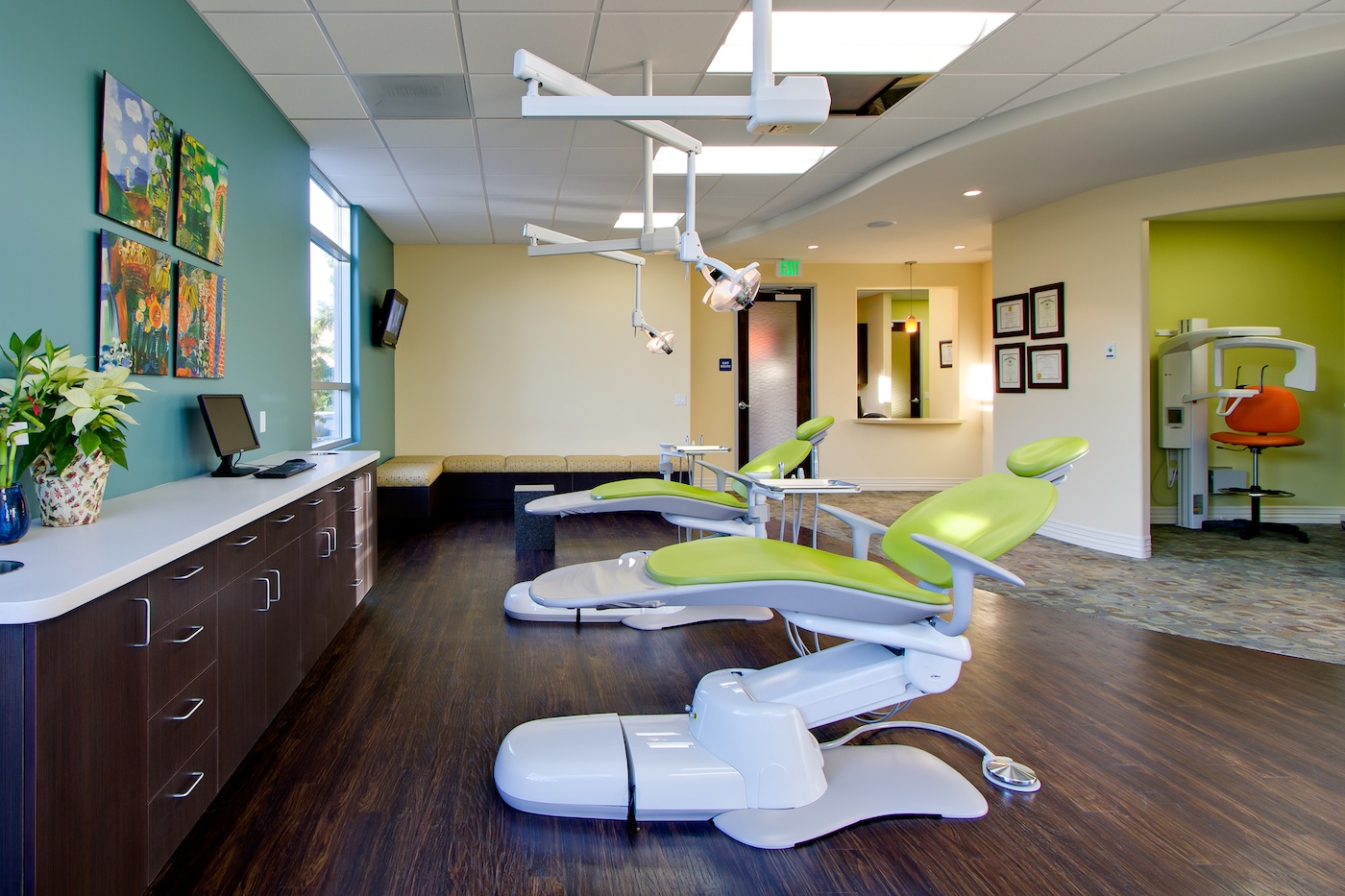This horizontally aligned rectangular image captures a modern, spacious dental office featuring two futuristic dental chairs with white bases and lime green cushions for the head, back, and seat. These chairs are equipped with reticulating arms ending in lights, suspended from the ceiling. The dark wood flooring extends throughout the room, contributing to the sleek aesthetic. On the left side, cabinetry with stainless steel handles and a white countertop is arranged beneath a green wall adorned with four square canvas prints. 

A small computer monitor is placed on the countertop, next to a keyboard, mouse, and a vase filled with flowers. Positioned against a pale yellow wall in the background, a cushioned bench for waiting patients is visible along with a frosted glass door. Another room is accessible via an archway on the right, characterized by brighter green walls and white baseboards. This adjacent space houses an orange swivel chair and a large piece of white equipment resembling a head x-ray machine.

Accreditation certificates are framed on the far right wall, while a reception area and a large window that allows natural light to spill in are also present in the background, creating a welcoming atmosphere.